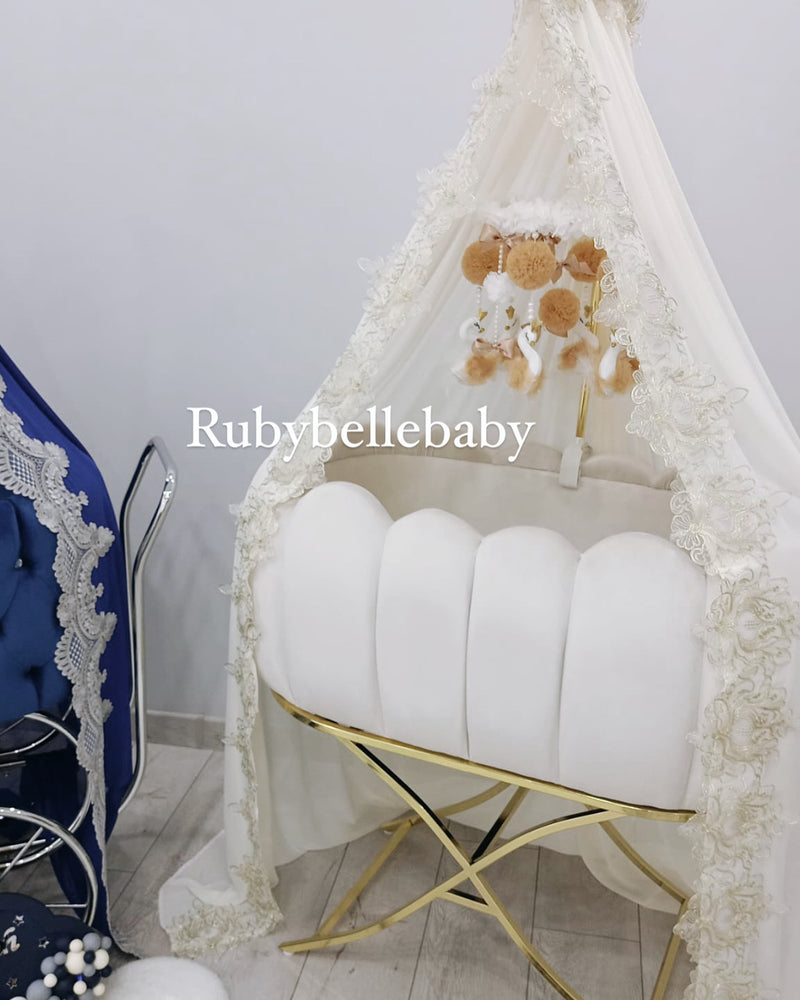This detailed photographic image presents an intricate indoor baby nursery scene. Central to the composition is a luxurious golden metal crib with distinctive X-shaped legs. The crib, which resembles a bassinet style, is adorned with four upright white pillows or cushions that line its sides like a picket fence, enhancing its plush appearance. Suspended above the crib is a delicate white lace curtain, draping down from the ceiling in a V or tent-like fashion, adding an ethereal touch to the setting. A whimsical mobile featuring brown and white ducks, as well as fuzzy brown pom-poms, hangs over the crib, providing a charming focal point for an infant. To the left of the crib stands an elegant old-fashioned baby carriage in blue, with a silver handle and silver-colored wheels. The entire scene is set on a polished hardwood floor, with the background featuring a white wall, likely within a well-appointed baby's room. Central in the image is the watermark text, "Ruby Bell Baby," in white, completing the serene yet sophisticated ambiance of the nursery.